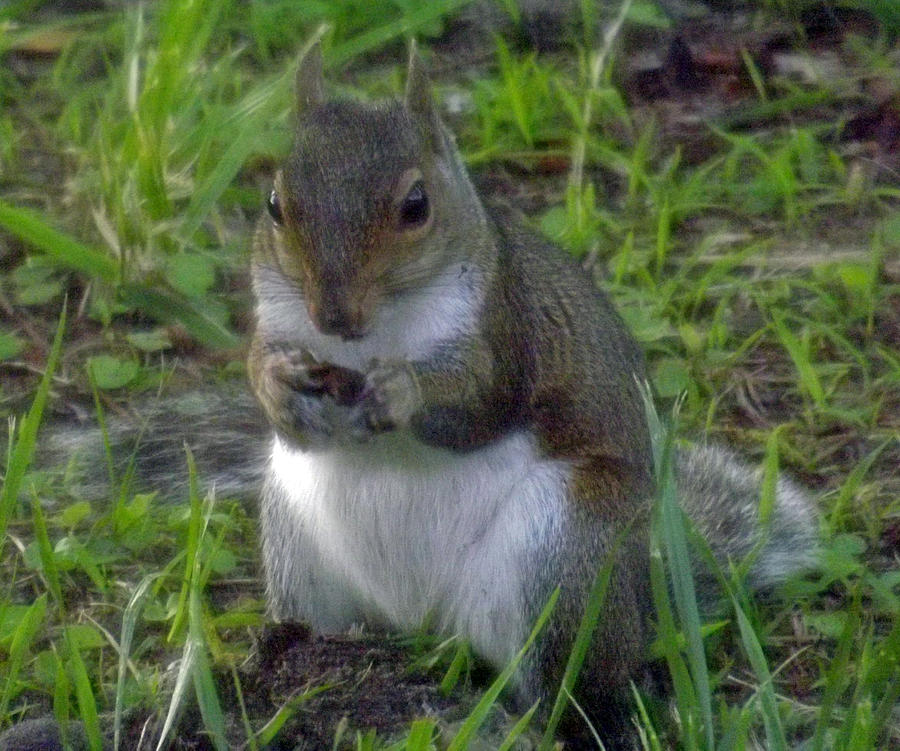This detailed image depicts a charming squirrel seated on a patch of brown soil, surrounded by green blades of grass and clover. The squirrel is intently nibbling on a round, brown acorn held delicately in its grayish-brown paws. Its prominent, bushy tail, colored shades of gray, white, and black, curves behind it, accentuating the soft fur that seems to blur into the earthy ground beneath. The squirrel's fur is primarily a blend of gray and brown, with a contrasting white belly that highlights its plump, well-fed appearance. Its face, heart-shaped and expressive, features keen, almond-shaped dark eyes that glisten with a hint of vigilance, long black whiskers, and upright ears. The background, slightly blurred, adds an almost painterly quality to the realistic depiction, making the squirrel the clear focal point as it gazes directly at the camera, seemingly protective of its prized acorn.